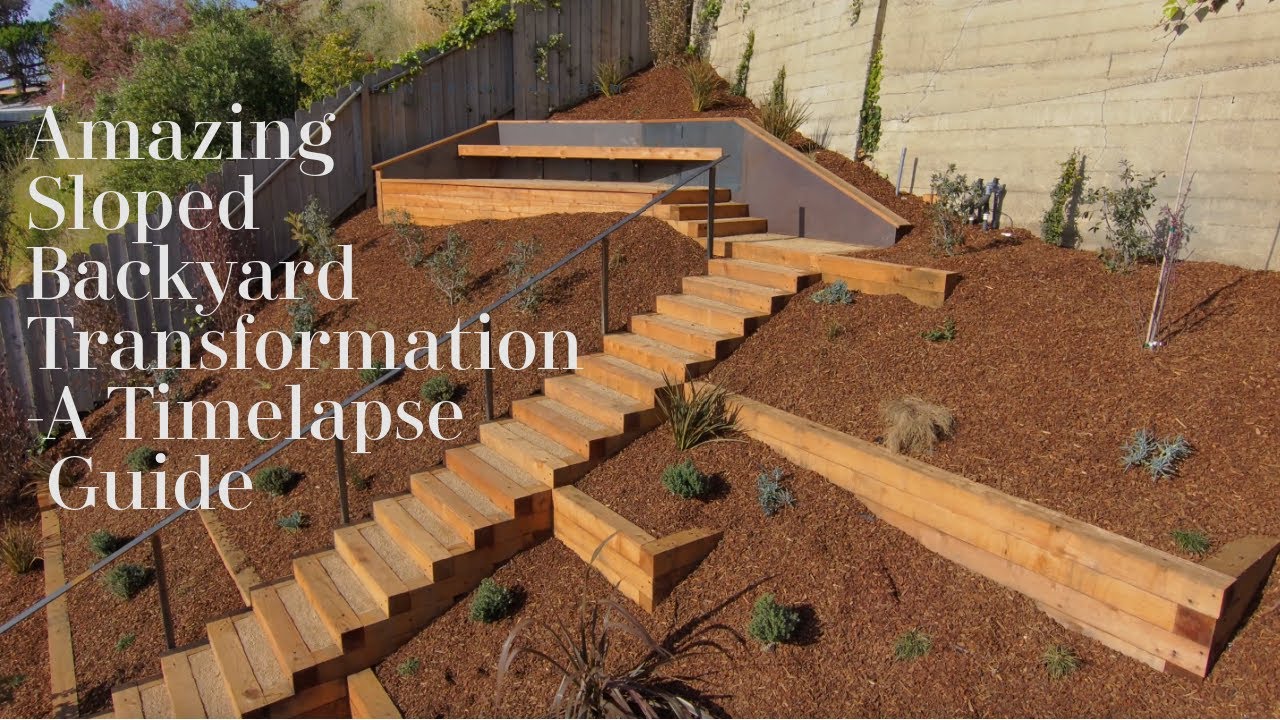The image appears to be the front page of an online instructional guide, such as a website, YouTube channel, or PowerPoint presentation, titled "Amazing Sloped Backyard Transformation: A Time-Lapse Guide." The photograph showcases a beautifully terraced backyard situated on a steep hill. The landscape features multiple wooden steps running up the middle, leading to a wooden seating platform or bench at the top. The entire area is covered in brown mulch, and various wooden boxes function as retaining walls for the terraced sections that facilitate vertical planting. Wooden fences enclose the yard, with a concrete wall and additional fencing visible in the background. Shaded by the sun, you can see the shadows cast by the interspersed plants, giving the scene a layered, textured appearance. This well-organized landscaped yard highlights a mix of natural beauty and structural ingenuity, creating a practical yet aesthetically pleasing outdoor space.